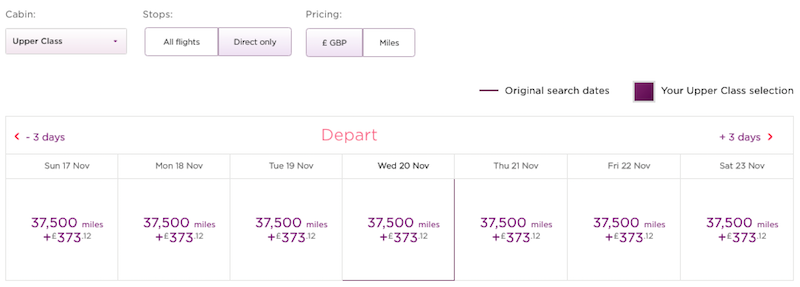The website displays information about booking flights, particularly highlighting an "Upper Class" cabin option. At the top of the page, there is a navigation bar with generic headings. Key information at the top includes options for direct flights, pricing in British Pounds, and the number of miles required for booking. These options are displayed within purple and white boxes, with grey-colored text and a delineating purple line for original search dates. 

In the main section, there is a large box indicating departure options. The box prominently features the word "DEPARTURE" in pink letters and provides options for departure dates categorized into "Less than 3 Days" on the left and "3+ Days" on the right. Below this, individual dates are listed, starting from Sunday, November 17th to Saturday, November 23rd. A darker line highlights Wednesday, November 30th.

For each date, the website shows a standard cost of "37.5 miles plus £373", consistently for each day listed. The miles required are displayed in purple, and the cash equivalent amount is also highlighted in purple boxes, assuring that the amounts remain constant across all dates. This indicates that the fare and miles required do not fluctuate for the given dates.